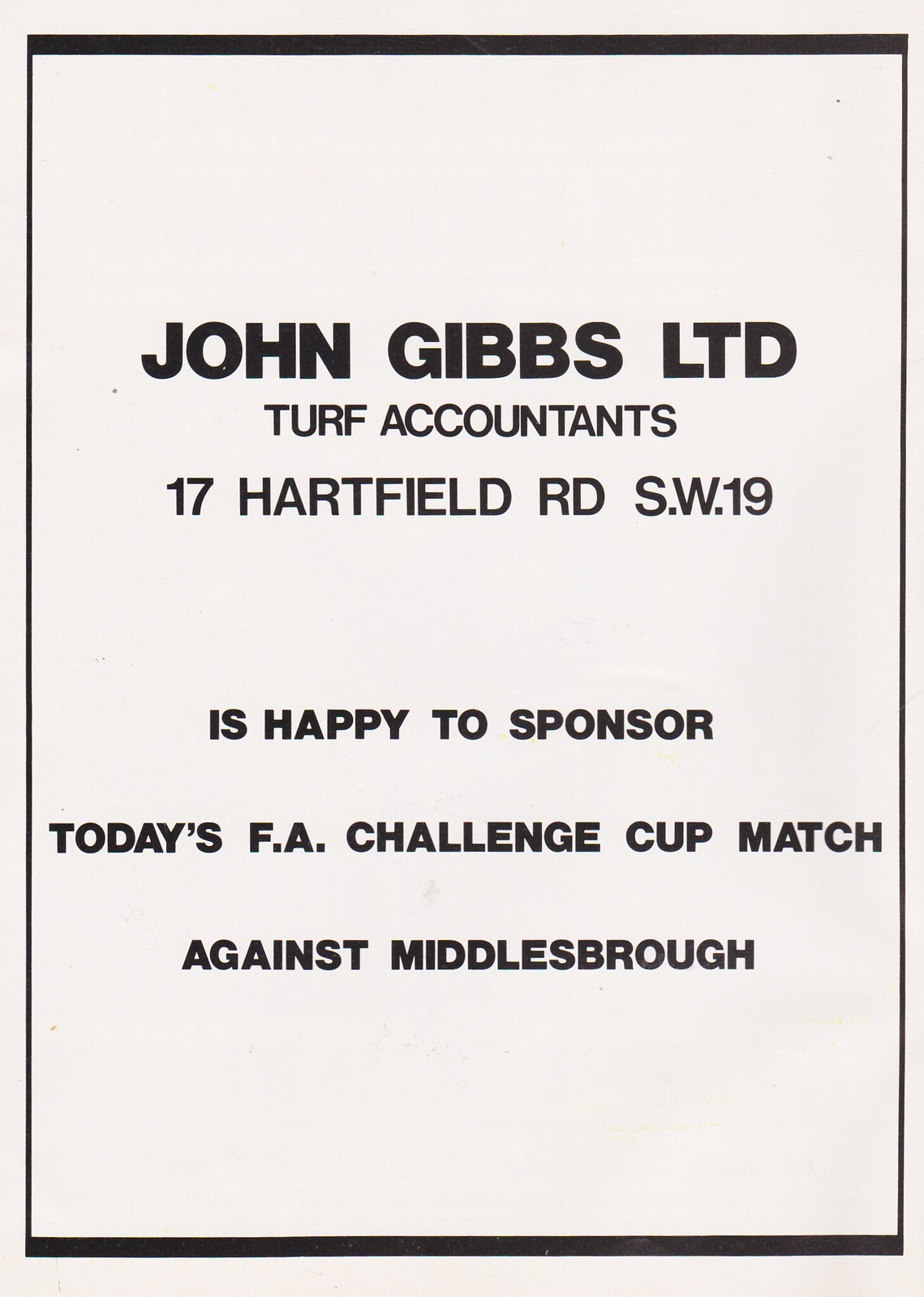The image displays a beige sign with a black outline about an inch from the edges, effectively centering the text within the bordered area. The top line features "John Gibbs Ltd" in bold, all-capital black text. Directly beneath it, in slightly thinner all-capital letters, are the words "Turf Accountants." The address "17 Hotfield Road, South West 19" follows, formatted in slightly larger lettering. Below the address, three lines of bold, all-capital text reveal the message: "HAPPY TO SPONSOR TODAY'S," "TODAY'S FA CHALLENGE CUP MATCH," "AGAINST MIDDLESBROUGH." The blocks of text are vertically justified, occupying the entire space within the sign, creating a balanced and organized appearance. The sign itself takes up the entirety of the image, which appears to be a sponsor advertisement for a game, all in the colors tan and black.